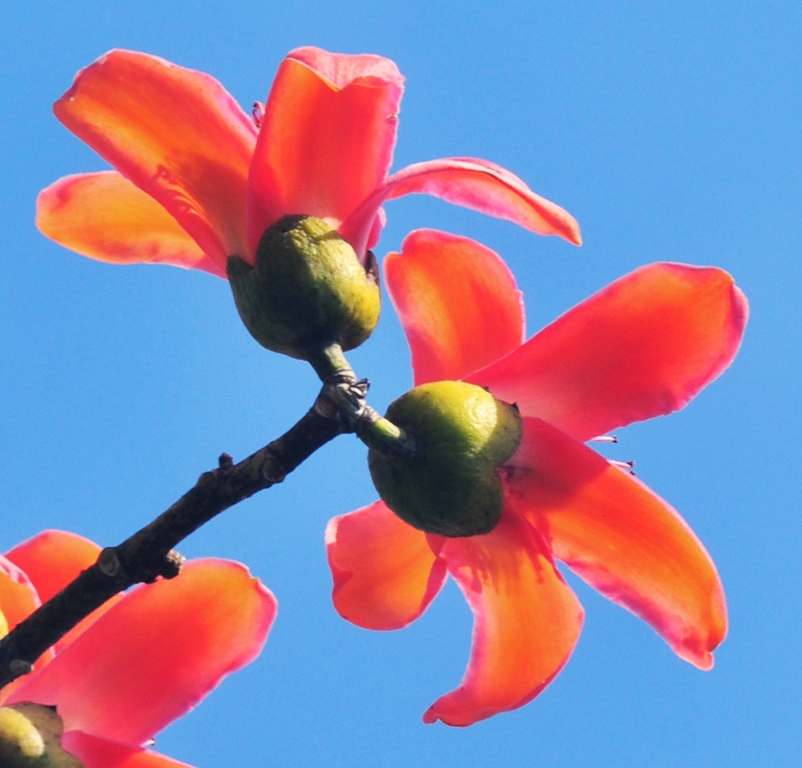This detailed photograph captures the striking beauty of a flowering plant against a clear, bright blue sky, evoking a sense of a sunny spring day. The image is taken from a low angle, as if the photographer is lying on the ground, aiming the camera upwards. The flower, perched on a green stem, boasts three individual blooms. Two of these flowers are prominently visible, displaying electric peach-colored petals, with hints of red and orange hues blending into each petal. These petals, numbering five on each bloom, possess an elongated, slender shape reminiscent of human tongues, gracefully radiating from dark green circular buds. The third bloom, partially visible in the bottom left, adds depth to the composition by peeking into the frame. The stem arches from the lower left to the center of the image, forming a Y shape where it splits into the two main blooms. The sky behind provides a smooth, cloudless backdrop, enhancing the vibrant colors of the flowers and emphasizing the bright, powerful sunlight of either morning or afternoon.